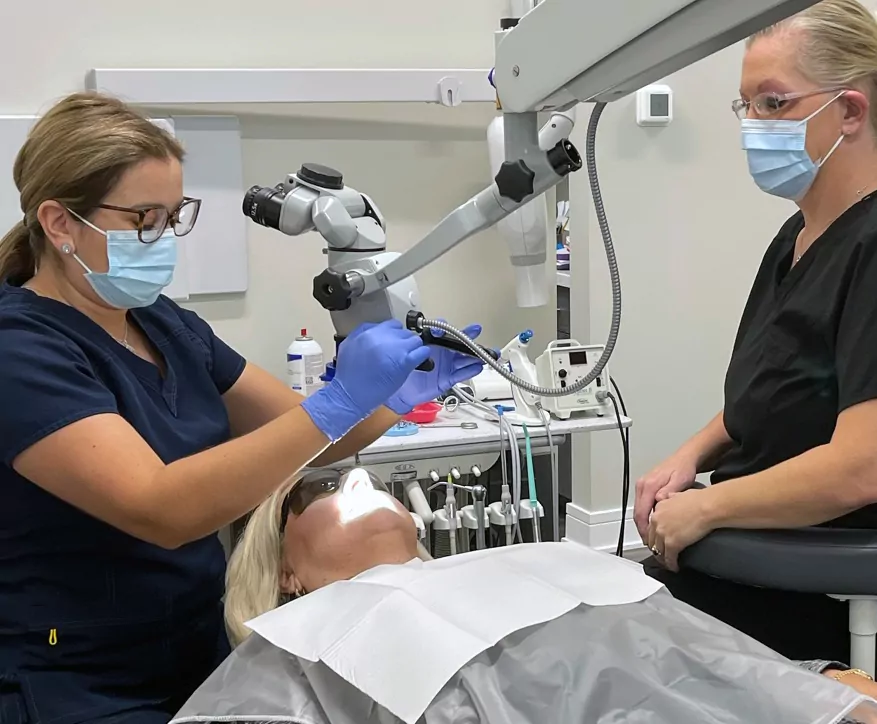The photograph captures a detailed scene in a bustling dentist office. A patient with loose, blonde hair is reclined in a dental chair, wearing dark sunglasses to protect her eyes from a bright light being used during the procedure. She is covered with a plastic smock and a paper bib across her chest. Two women, likely dental professionals, are attending to her. Both the women have sandy-colored hair, are wearing surgical masks, glasses, and scrubs—one in black and the other in navy blue. The professional in navy blue is adjusting a piece of equipment on a boom arm, which is positioned above the patient's open mouth and emitting a bright light. The professional in black scrubs is observing closely. Various dental instruments and equipment are visible in the background, hinting at a potentially complex procedure such as teeth whitening, cleaning, or other dental treatment being performed. The atmosphere is clinical and methodical, highlighting the meticulous nature of dental care.